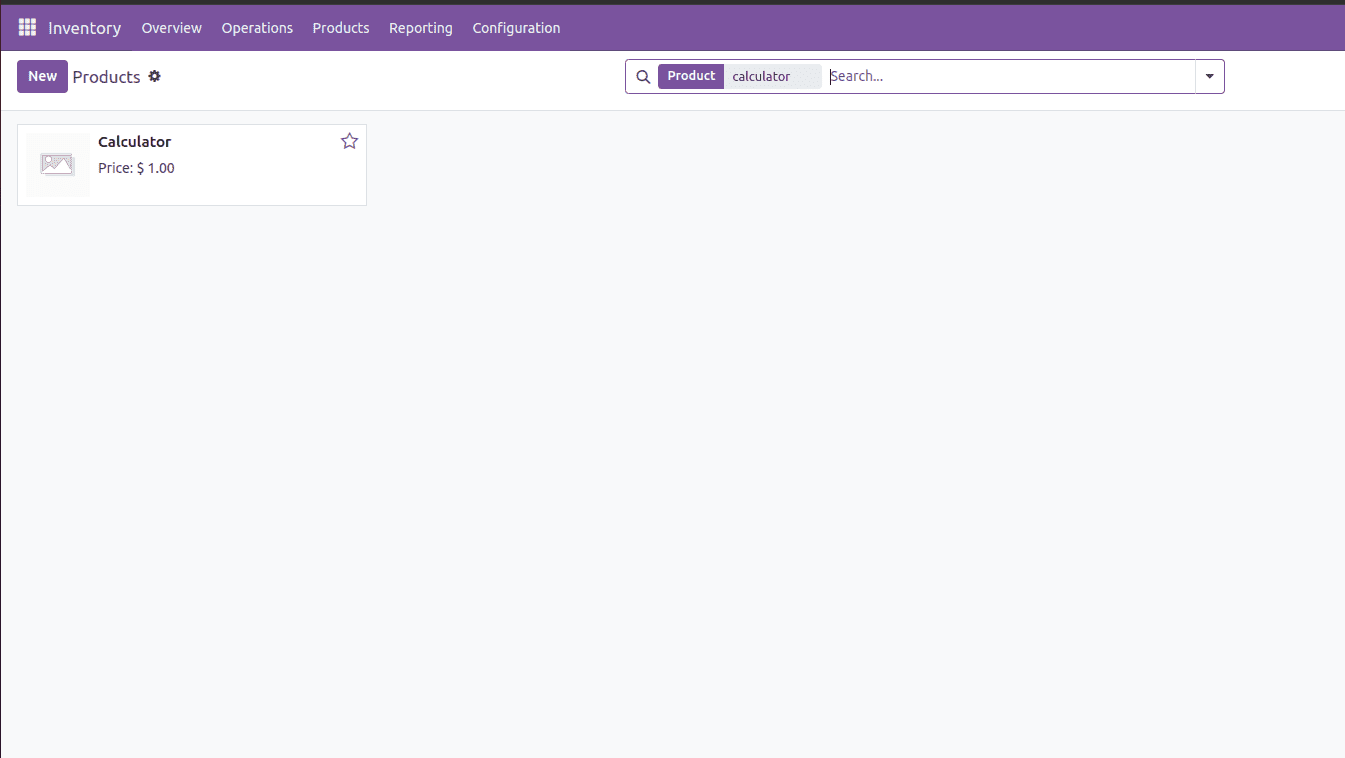This screenshot showcases a minimalist webpage interface. At the very top, a purple navigation bar spans across the page. In the upper left corner, an array of nine small white cubes is displayed, followed by the word "Inventory" in a white font. To the right of "Inventory," the following options are listed in the same white font: "Overview," "Operations," "Products," "Reporting," and "Configuration."

Directly beneath this navigation bar, a large white rectangular section serves as a secondary header. On the left side of this section, a purple square with the label "New" in white font is positioned. Next to it, "Products" is displayed in a bold black font, accompanied by a small gear icon to its right. Adjacent to the header, there is a search field with a black outline.

The search field contains two buttons inside it: the "Product" button, which is purple, and the "Calculator" button, which is gray. A small black magnifying glass icon is situated within the search field, which contains the placeholder text "Search..." indicated by a blinking cursor. At the right end of the search field, there is a downward-pointing arrow icon signaling the availability of a drop-down menu.

The main body of the webpage has a solid gray background. In the upper left section of this gray area, a white rectangular box is displayed with the word "Calculator" inscribed in black font. In the top right corner of this box, there is a little five-pointed star icon. Beneath the icon, the price "$1.00" is prominently displayed in black font.